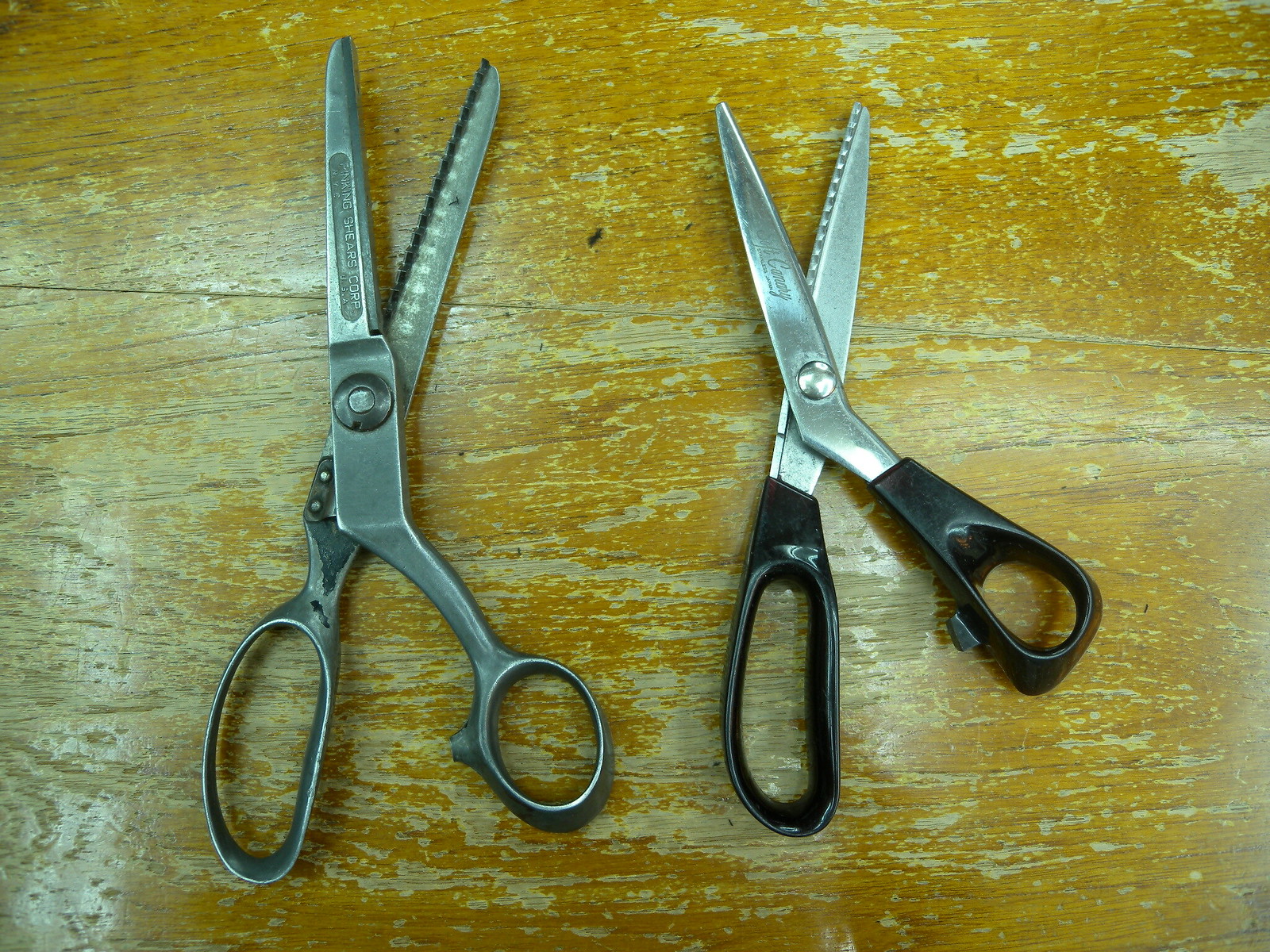This image captures two pairs of fabric-cutting scissors lying on a heavily distressed wooden surface, possibly a worn-out table or desk. The surface is significantly scratched and its lacquer has faded, revealing the aged, dry wood beneath. The pair of scissors on the left is entirely gray, with a slightly darker handle, and is the larger of the two. Both pairs of scissors are partially open, displaying angular toothed edges typical for cutting fabric. The smaller scissors on the right feature black plastic handles and metal cutting shears. Both pairs bear some unknown brand name etched into the metal, though the print is too small to decipher. The scissors and the setting together evoke a sense of long use and age.